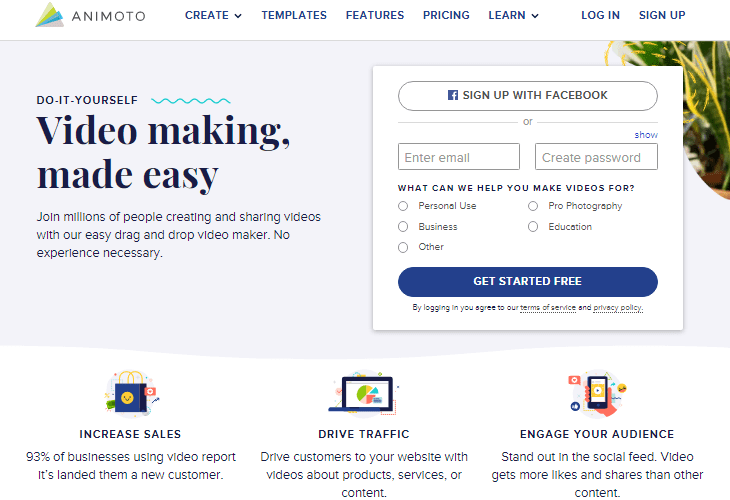The top left of the image features a triangle icon. Adjacent to it are menu options labeled "Model, Create, Templates, Features," hinting at various tools or functionalities available on this platform. There is a gray square button labeled "Do it yourself." Below this, a dynamic blue squiggly line curves across the image, accompanied by the slogan, "Video making made easy. Join millions of people creating and sharing videos with an easy drag and drop video maker, no explanation necessary."

In the top right, a patch of grass can be seen under a white bar prompting users to "Sign up with Facebook," or alternatively, enter their email and create a password. Below this, the question "What can I help to make videos for?" is posed, addressing potential users such as business owners proud of their photography, or educational content creators. A prominent blue oval button reads "Get started free," with a note suggesting users need to agree to the terms and service and privacy policy.

To the left side of the image, a section highlights increasing sales, illustrated with a bag icon. It states, "93% of businesses using video report it has landed them new customers." Below, the importance of driving traffic is emphasized. Various colored icons (green, yellow, blue, pink, red) representing a laptop and other tools suggest that videos for products, services, or content can attract customers to one's website. Towards the bottom, an image of a phone underscores audience engagement, with a note stating, "Stand out on the social feed, video gets more likes and shares than other content."